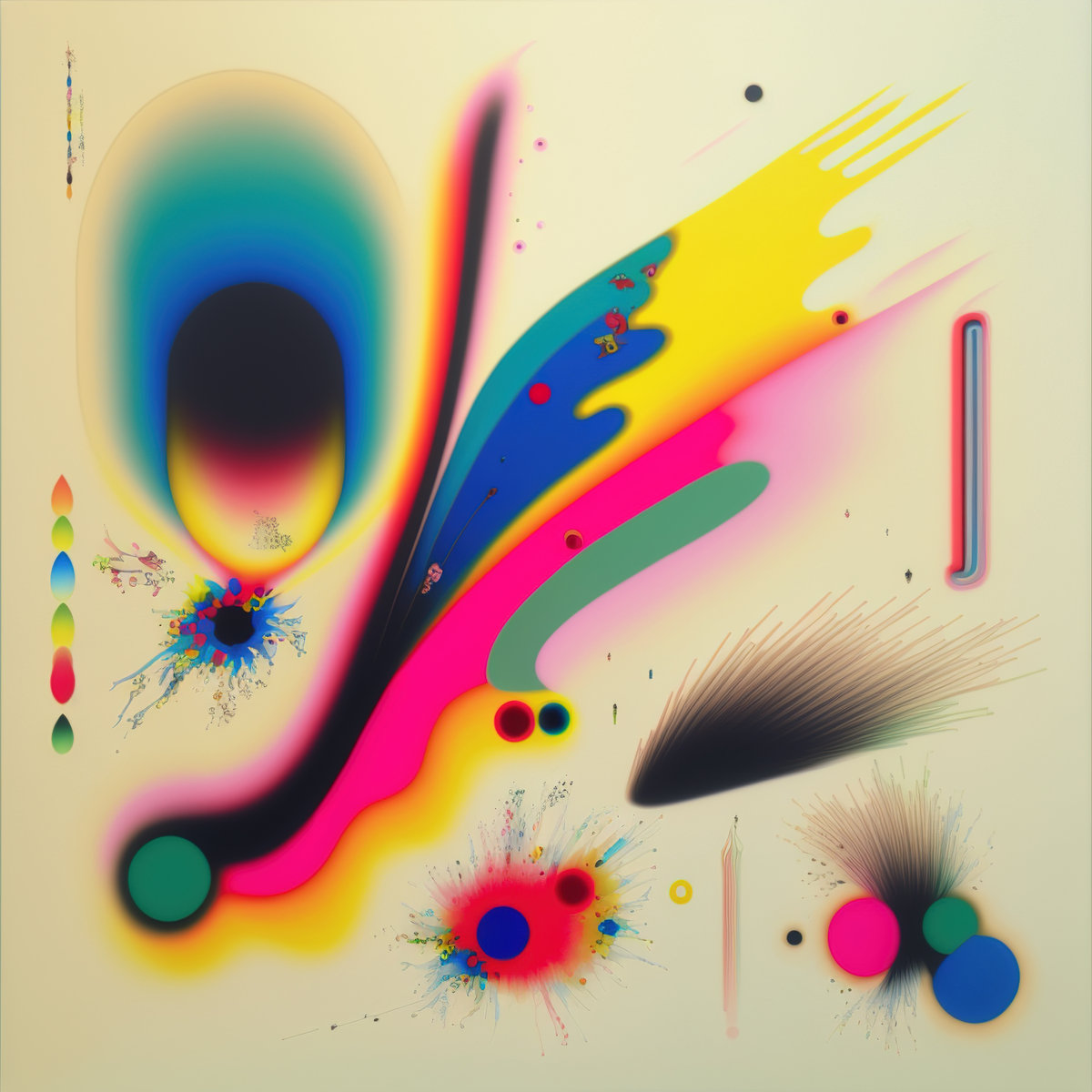This vibrant digital artwork features a striking composition of various neon colors against a beige-white, almost cream-colored background. The intricate piece showcases a variety of techniques suggesting an exploration of digital art tools. Dominating the center of the image is a long, flowing, multicolored splotch originating from a green dot in the lower left portion, with hues of pink, blue, yellow, green, black, and light blue extending towards the upper right corner. The top left area bursts with shades of blue, dark purple, orange, and yellow, transitioning into a splatter of dark purple, blue, and magenta. Further down, another significant green dot emits dark purple, magenta, dark blue, aqua blue, and yellow streaks. The artwork also features gradient drips, airbrushed spots, and splattered paint effects, creating a dynamic assembly of circles, lines, and splotches in vibrant pinks, blues, yellows, and greens. This detailed piece encapsulates the experimental and expressive nature of modern digital art.